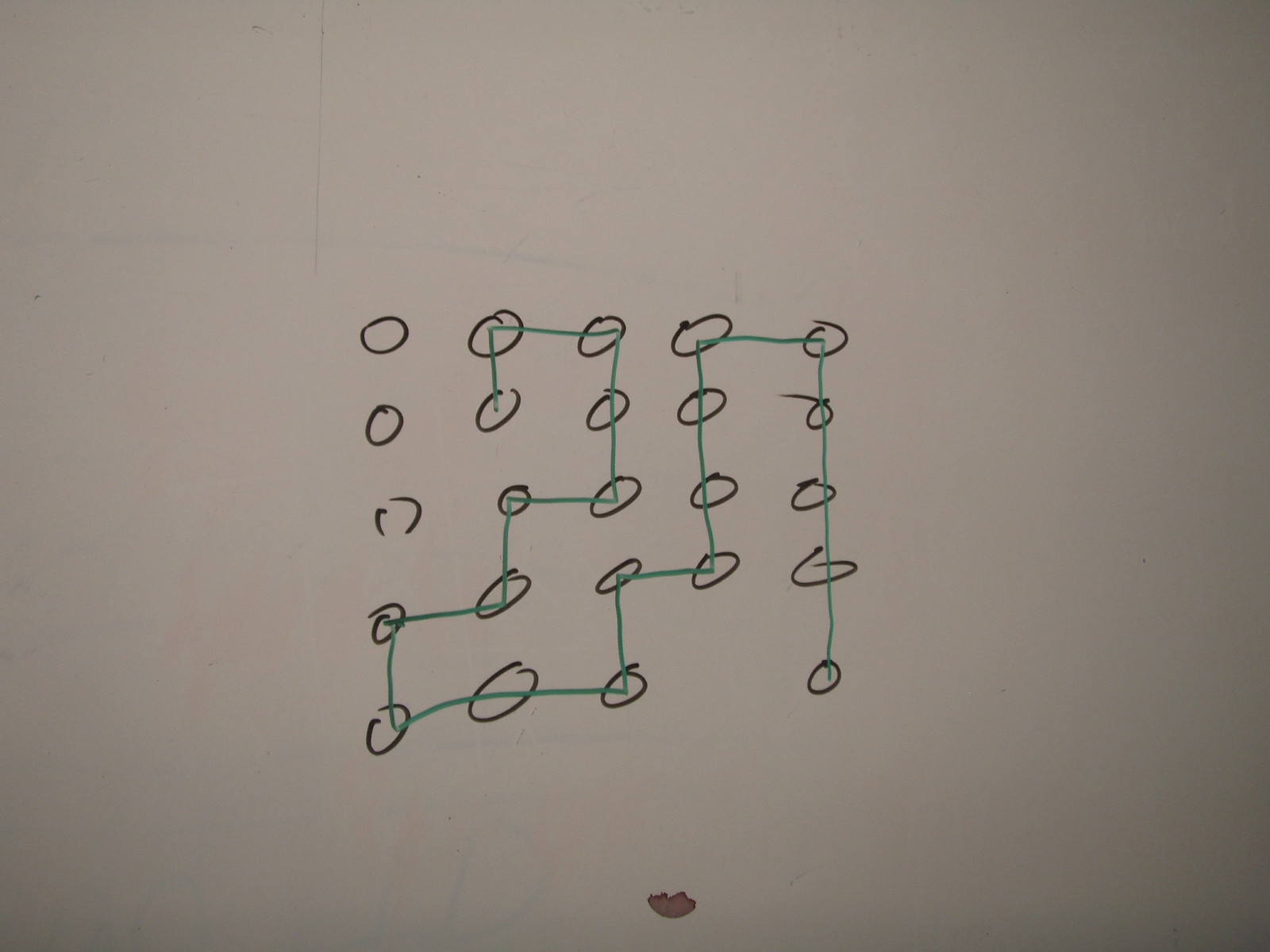The image appears to be a whimsical hand-drawn sketch on a piece of paper, primarily utilizing green and black markers. The paper itself shows signs of wear and distress, with a noticeable brownish stain or possible tear towards the bottom center. This stain gives the appearance of either a rip in the paper or a coffee stain.

The sketch is intricate yet chaotic, with a series of hand-drawn circles, predominantly in black, arranged in a seemingly 5-by-5 grid, though one circle is conspicuously missing. Within the top-left quadrant of the drawing, there are faint marks and lines. These black circles vary slightly in shape and neatness, indicating a freehand drawing style.

Interconnecting these black circles is a zigzagging green line that moves erratically across the page. The line starts by connecting three vertically aligned circles before continuing with an unpredictable pattern, tracing a path that meanders to the right, then up, right again, and up again, before heading left and continuing in this uneven manner. This green marker line runs through the center of the circles and adds a layer of dynamic movement to the scene.

The rest of the page remains blank, with the paper color being either white or slightly off-white, enhancing the focus on the central chaotic drawing and the contrasting colors.